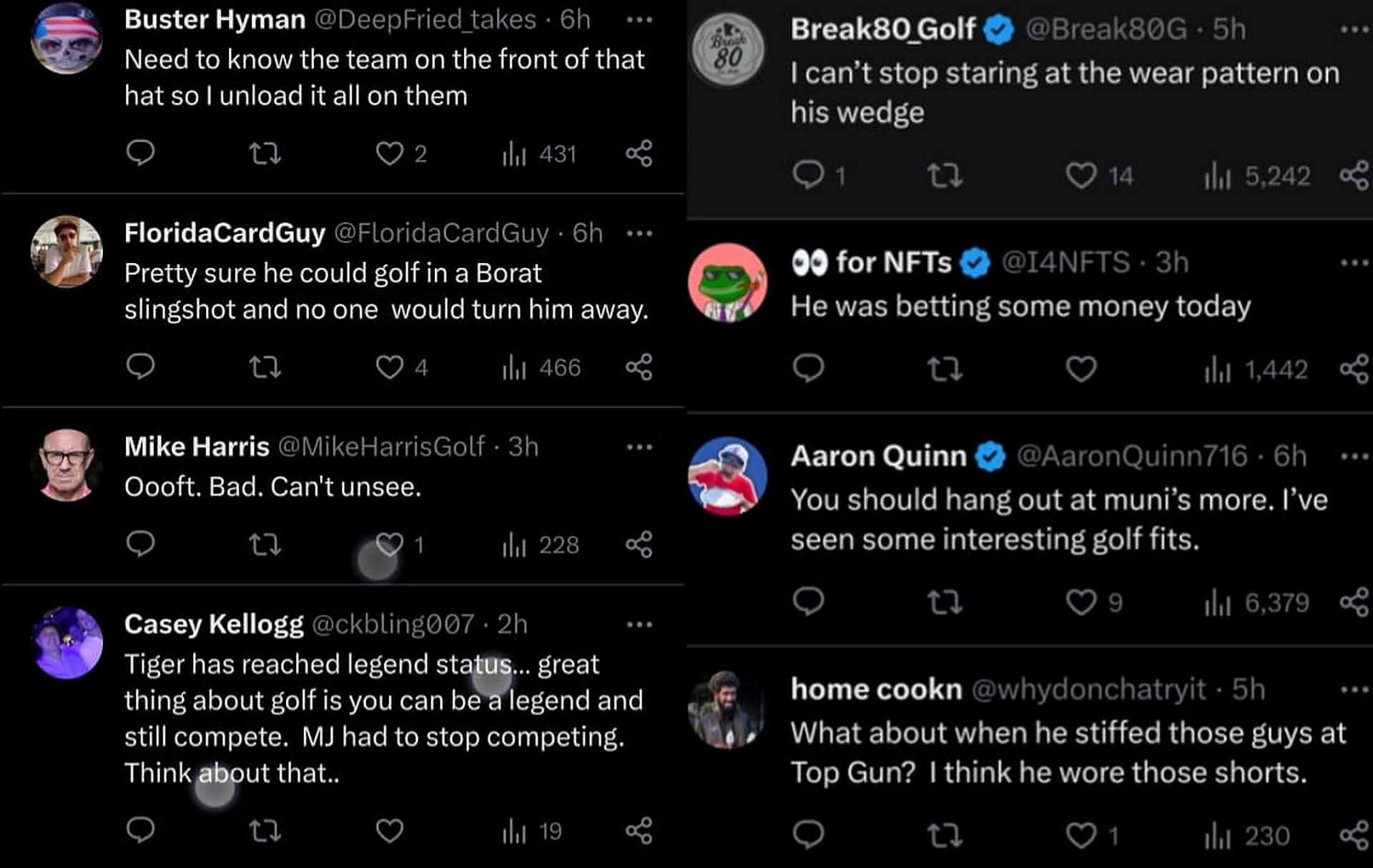A detailed caption for the image could be:

"A screenshot showcasing multiple responses to a social media post, with a black background and white text for names and comments. Each commenter has a profile picture icon next to their name. On the left side, four comments are displayed vertically: 

1. Buster Hyman: 'Need to know the team on the front of that hat, so I unload it all on them.'
2. Florida Card Guy: 'Pretty sure he can golf in a Borat slingshot. No one would turn him away.'
3. Mike Harris: 'Oofed, bad, can't unsee.'
4. Casey Kellogg: 'Tiger has reached legend status. Great thing about golf is you can be a legend and still compete. MJ had to stop competing. Think about that.'

On the right side, four more comments are vertically aligned:

1. break80_golf: 'I can't stop staring at the wear pattern on his wedge.'
2. Eyeballs for NFTs: 'He was betting some money today.'
3. Aaron Quinn: 'You should hang out at Mooney's more. I've seen some interesting golf fits.'
4. homecooking: 'What about when he stepped those guys at Top Gun? I think he wore those shorts. Must be talking about Tiger Woods.'

Each comment provides a unique perspective, blending humor and insight into the conversation thread."